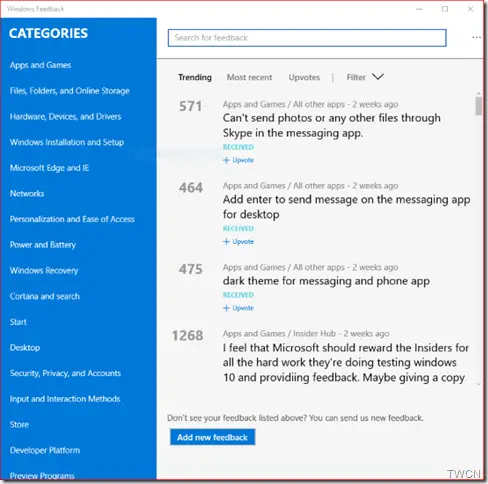This web page serves as an interface for Windows Feedback. At the top, a red banner prominently displays the title "Windows Feedback." Below the banner, the page is divided into several sections, each aiming to facilitate user interaction and feedback submission.

On the left side is a list of categories, each written in white letters and set against a blue background. The categories include: 

1. Apps and Games
2. Files, Folders, and Online Storage
3. Hardware, Devices, and Drivers
4. Windows Installation and Setup
5. Microsoft Edge and IE
6. Networks
7. Personalization and Ease of Access
8. Power and Battery
9. Windows Recovery
10. Cortana and Search
11. Start, Desktop
12. Security, Privacy, and Accounts
13. Input and Interaction Methods
14. Store
15. Developer Platform
16. Preview Programs

The word "CATEGORIES" is prominently displayed at the top of this section in bold, capitalized white font. 

To the right of the categories is a search bar, framed by a blue border, which allows users to "search for feedback". 

Below the search bar are options to filter feedback by what's "Trending", "Most Recent Upvotes", etc., with "Trending" displayed in bold.

The feedback entries begin with various issues and suggestions from users. Some examples include:

- *Apps and Games, All Other Apps, two weeks ago*: "Can't send photos or any other files through Skype in the messaging app."
- *Apps and Games, All Other Apps, two weeks ago*: "Add enter to send message on the messaging app for desktop."
- *Apps and Games, All Other Apps, two weeks ago*: "Dark theme for messaging and phone app."
- *Apps and Games, Insider Hub, two weeks ago*: "I feel that Microsoft should reward the insiders for all the hard work they're doing, testing Windows 10 and providing feedback, maybe giving a copy."

At the bottom of the feedback list is a prompt for those who don't see their feedback listed above, encouraging them to send new feedback. A prominent button with a blue background and white text invites users to "Add New Feedback."